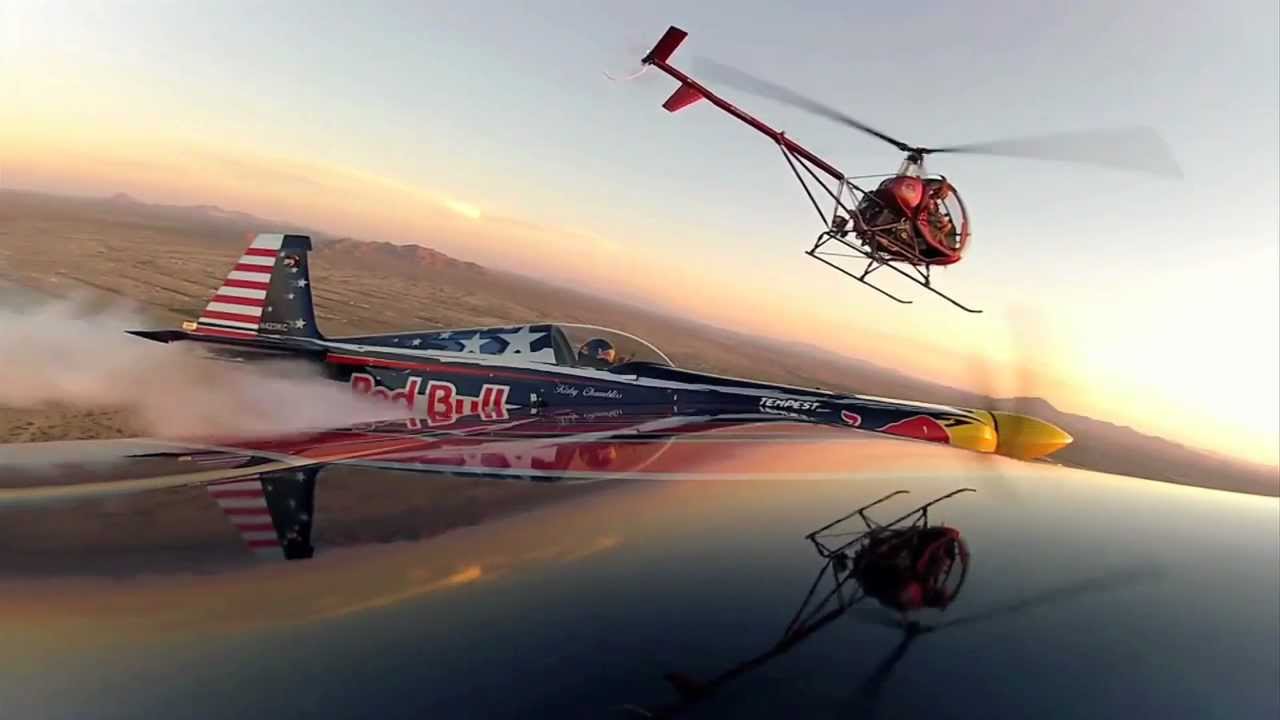This captivating image features a vibrant Red Bull racing jet in mid-flight, adorned in striking red, white, and blue colors. The jet's sleek design includes a yellow propeller and pointy yellow nose. The Red Bull logo, prominently displayed in red letters against a white backdrop, is visible right behind the pilot, who is seen wearing a helmet inside the cockpit. The jet leaves a trail of white smoke as it speeds through the sky. Above the jet, a red helicopter, equipped with skis and a visible propeller, hovers closely. The helicopter’s reflection can be seen in the water below, enhancing the scene's dynamic composition. The background showcases a flat, desert-like horizon with rock formations, possibly in a southwestern region like Arizona or California. The sky displays a soft gradient of oranges and pinks, indicating either sunrise or sunset, adding a warm glow to the impressive aerial display.